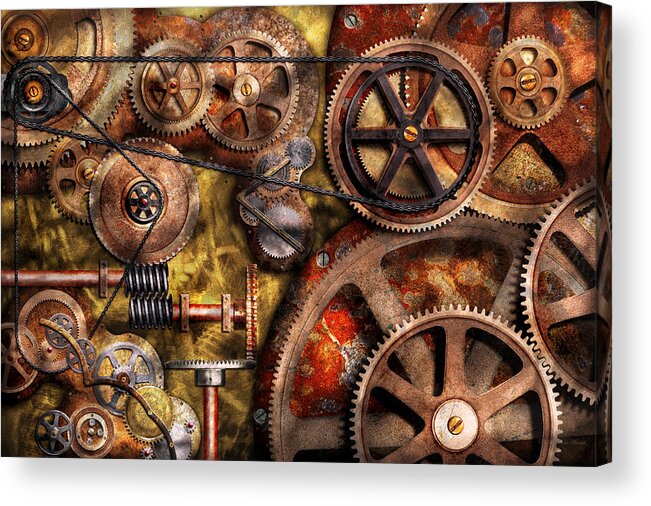The image is a detailed color painting depicting a complex array of interlocking gears and chains, forming a machine-like structure. Dominating the composition are a dozen or more gears of varying sizes and colors, including rusty brown, gold, copper, bronze, and black. 

At the top front, a large wheel with black steel spokes has a chain wrapped around it, extending to a smaller wheel, giving it a resemblance to a bicycle frame. The lower right corner features the largest gears, colored in a rusty brown hue with solid steel construction and wide spokes, further interlocking with surrounding gears. 

The right-hand corner showcases three sharp-toothed gears in a grayish tone. Just above these, a gold gear with red trim is connected to a bronze gear with black trim, which has a long chain that attaches to a small black gear located in the upper left corner of the image. 

In between these larger gears, several smaller bronze gears are set against a weathered, yellow-toned background. Additionally, the bottom left corner houses a cluster of tiny gears, while nearby, a few pipe-like objects with black covers add to the intricate mechanical aesthetic. The overall impression is reminiscent of the inner workings of an antique clock or a vintage music box, with an old and rusty ambiance that suggests age and wear.